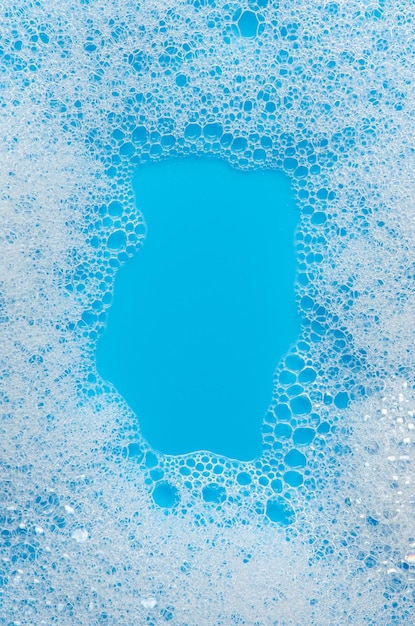This image is a close-up of a soapy, light blue surface, likely taken from above. The center of the image reveals a bright sky blue floor, which is exposed in an irregular shape amidst the surrounding soap suds. The borders of the image are dominated by a thick layer of white foam, while the middle showcases a nearly rectangular but unevenly shaped clear area free of bubbles. The bubbles themselves vary in size; larger, more transparent bubbles are found closer to the center, gradually becoming denser and whiter as they spread outward. The light blue underneath suggests either a bathtub or a sink filled with soapy water. No other objects or text are present, focusing purely on the interplay between the clean blue surface and the frothy white bubbles. The image's close-up perspective creates a visually interesting, almost abstract scene with just two primary colors: light blue and white.